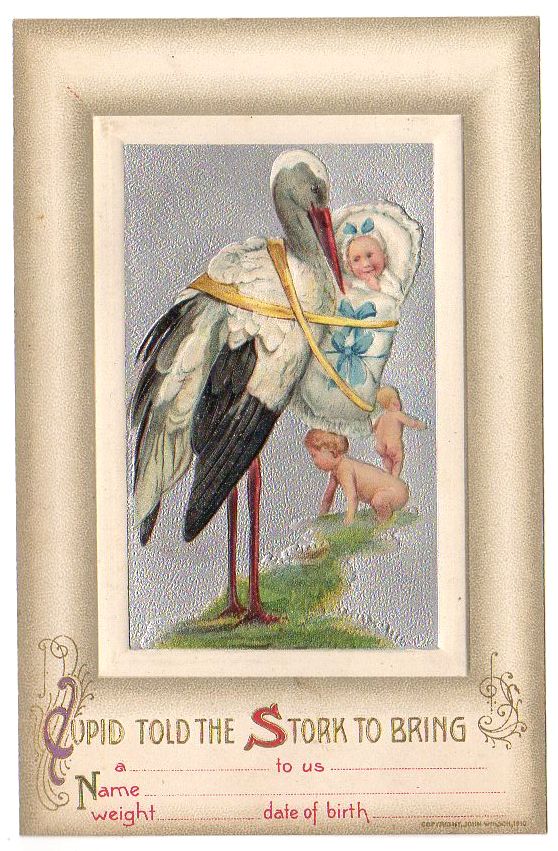The image depicts a vintage-style painting, likely from the early 1900s, designed as a baby announcement card. The central figure is a stork, characterized by its white plumage with black-tipped wings, a rounded white and gray head, and a long, pointed red beak. The stork stands on tall red legs and carries a baby in a white, fluffy bed-like contraption, secured with red tape. The baby, appearing Caucasian, is adorned with blue bows. Below the stork, two naked babies are playing in green grass against a speckled white background. The painting also has a beige outer frame. At the bottom, there is red text that reads, "Cupid told the stork to bring a [blank] to us," followed by empty lines for the baby's name, weight, and date of birth, allowing for personalization.